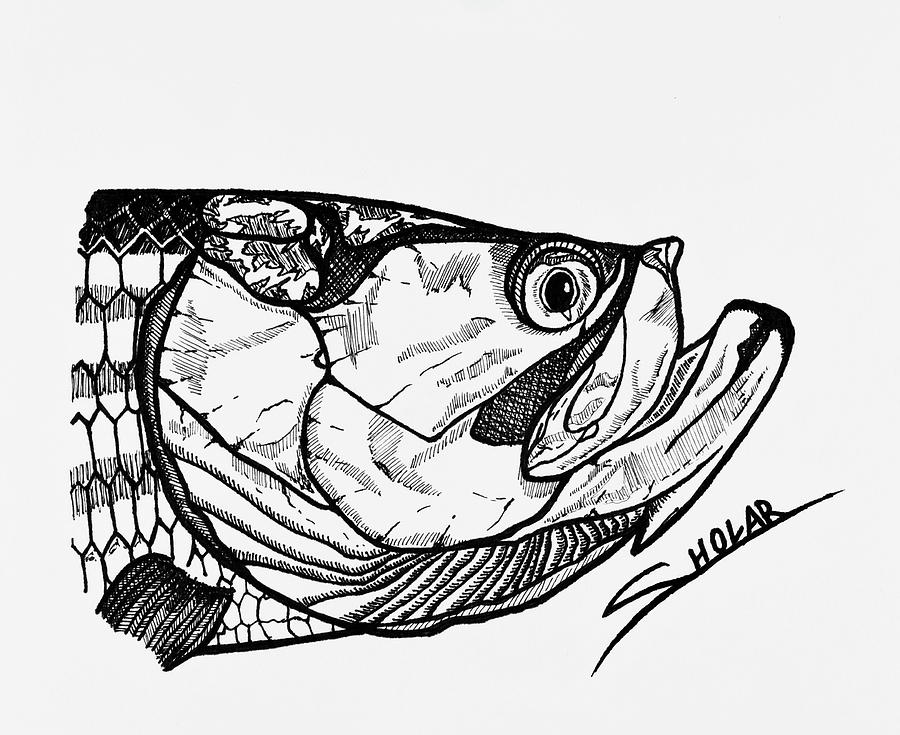This detailed black and white fine-lined drawing depicts a close-up side view of a fish head positioned against a very light gray background. The fish, which resembles a bass, features a prominent lower jaw that extends beyond the upper jaw and a pointed nose. Its large, round eye has a deep black center. The scales are intricately detailed, appearing rectangular with pointed tops and bottoms. The drawing captures the texture and structure of the fish's head, including the gill linings and the small front fin, visible at the bottom. The fish's mouth is slightly open, curving upwards. Written diagonally, curving up across the bottom right-hand corner of the image, is the word "H-O-L-R-A," with the "S" character stylized to underline the rest of the text.